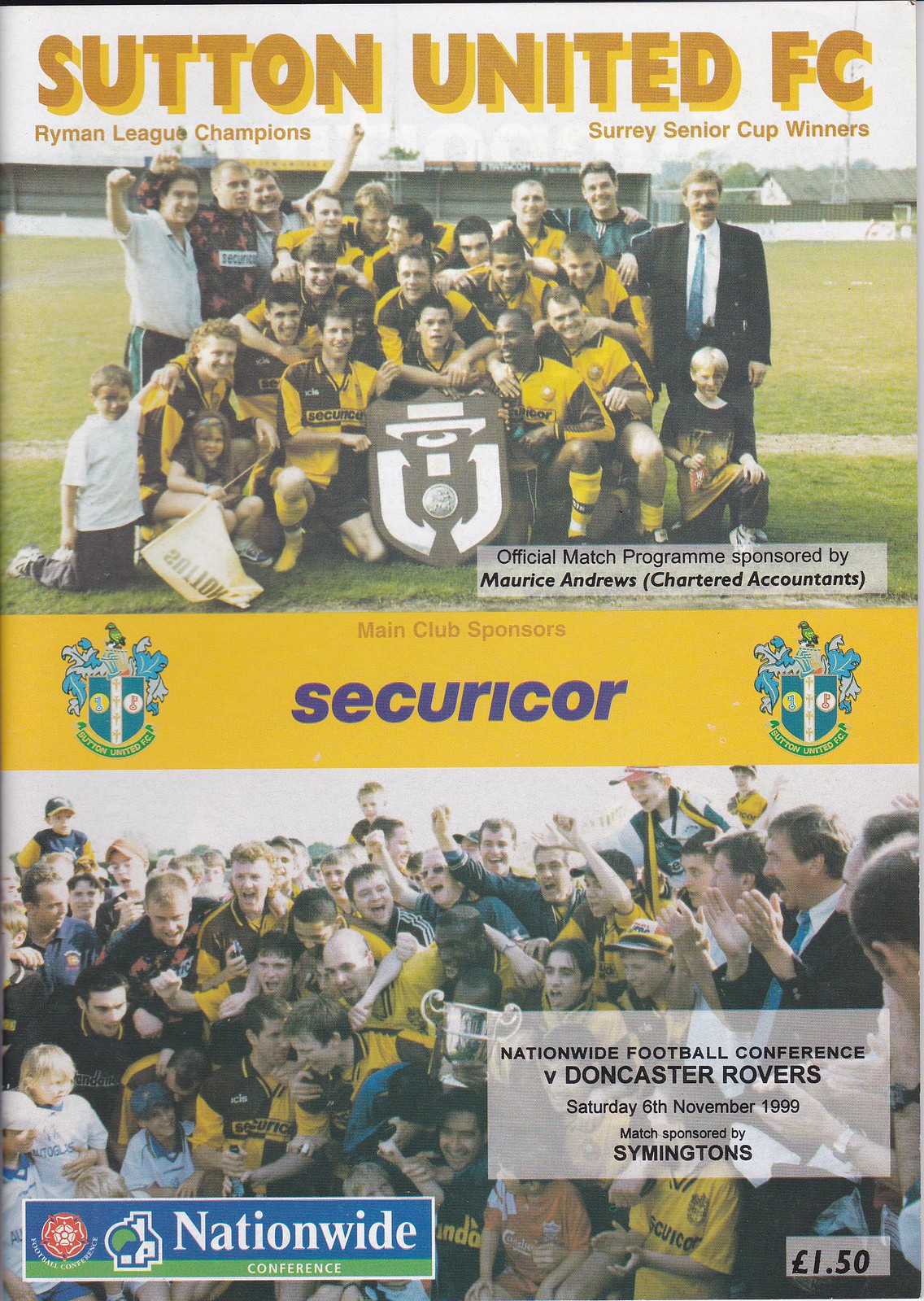The image displays the front page of a detailed publication associated with a sports event, specifically a match involving Sutton United F.C. The cover is divided into two main sections and features multiple elements. At the top, against a white banner, it reads "Sutton United F.C.," with the accolades "Ryman League Champions" on the left and "Surrey Senior Cup winners" on the right. Below this, there is a large photograph depicting the football team in yellow and black kits, posing together on a football pitch. The bottom right corner of this photo features the text "Official Match Programme sponsored by Maurice Andrews Chartered Accountants."

Beneath this section lies a prominent yellow banner stating "Main Club Sponsors Securicor." Below the banner, another large photograph is visible. This image showcases a more chaotic scene with the same yellow and black-clad team members celebrating amidst a sea of people, including children and adults. To the right of this packed scene, text notes "Nationwide Football Conference vs. Doncaster Rovers, Saturday 6th November 1999. Match sponsored by Symingtons." The bottom corners of the page respectively display the price of the publication at £1.50 in the bottom right and an advertisement for Nationwide in the bottom left. The overall color scheme prominently features yellow, black, red, and elements of blue or green for the logos.